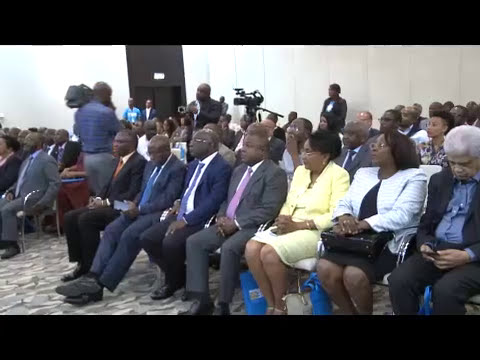The photograph depicts an indoor setting within a large meeting hall, characterized by white walls and a gray and white carpet. The audience comprises predominantly middle-aged to elderly African-American individuals, all clad in formal attire. The men wear suits and ties, while the women don dresses and jackets. Seated in rows of chairs, the individuals appear highly attentive, suggesting a serious event, possibly a political or prayer meeting.

The front row prominently features four black men in their 50s to early 60s, seated from left to right. Adjacent to them, moving rightwards in the image, are three black women: the first is in her 50s, dressed in a matching yellow dress and jacket; the second, in her 40s, wears a black dress with a white jacket, her hair elegantly styled, and she sports glasses; the third, a woman in her late 60s or 70s, wears gray slacks paired with a black jacket and a blue blouse, her head bowed in what appears to be either deep thought, prayer, or sleep. The women have their hands folded in their laps, their legs crossed at the ankles, while the men rest their hands relaxed over their laps.

The room includes more rows of people in the background where detailed features are less distinguishable. A significant detail is a cameraman, positioned in the aisle on the left side of the image, holding a large video camera, reminiscent of those used in news productions. Additionally, a camera is installed on the floor to capture the event. The rear part of the room features a black door. Overall, the image exudes a sense of order and solemnity, reflective of the event taking place.